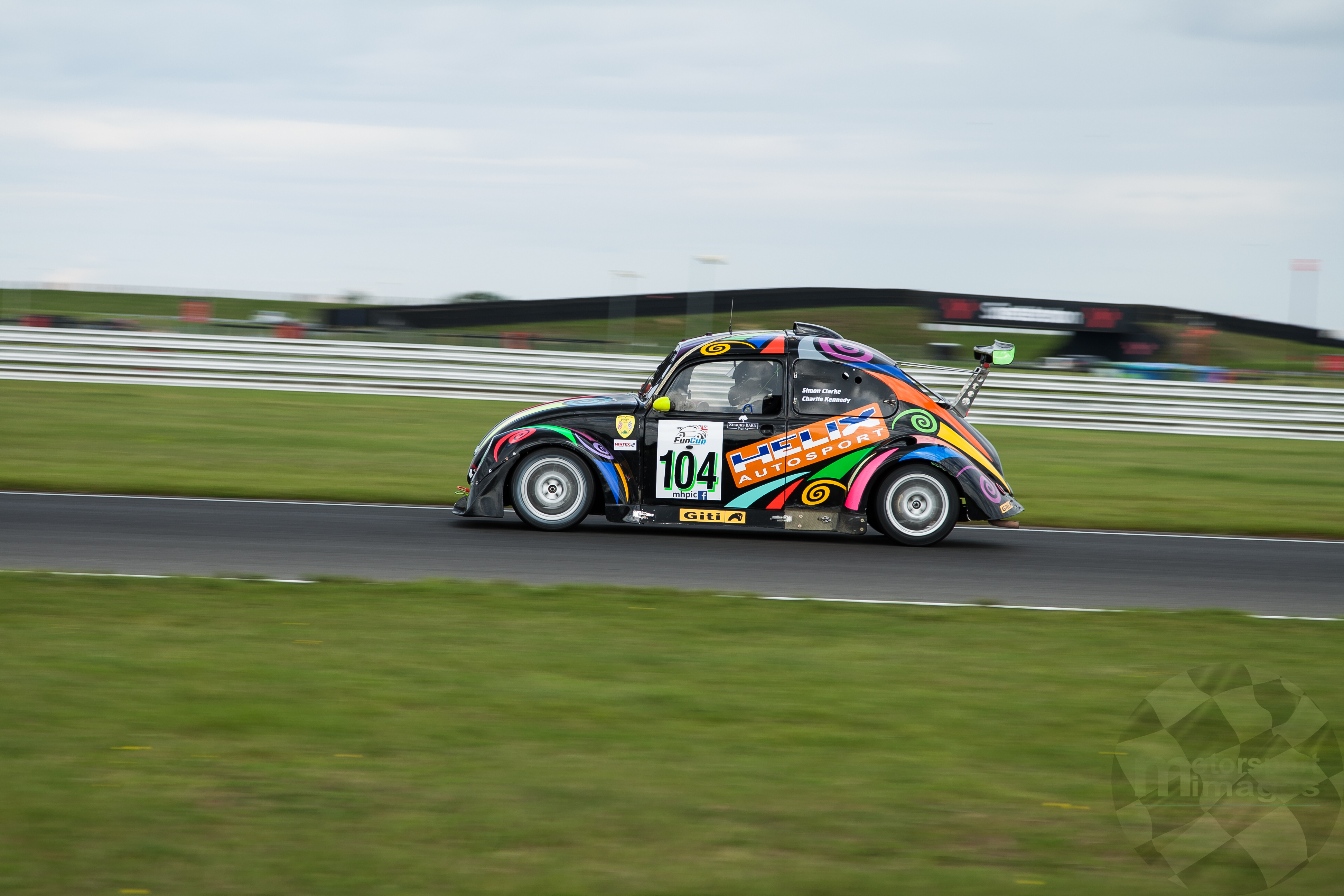This charming photograph captures a vintage 1970s Volkswagen Beetle Bug race car, adorned with a vibrant, multicolored paint job featuring an array of swirling lines and thick retro designs in hues of purple, hot pink, orange, green, turquoise, yellow, and blue. The car, primarily black, is embellished with a striking orange rectangular logo on the driver's door that reads "Helix Autosport" in blue and white letters. A prominent white square on the same door displays the number 104 in black. The vehicle is equipped with a spoiler on the back, adding to its sporty appearance. Inside, a race car driver wearing a black helmet can be seen. The Bug is actively racing on a black asphalt track, flanked by grassy areas and a white fence, with an overcast yet clear sky serving as the backdrop. This lively race scene not only showcases the car's unique aesthetic but also its dynamic presence on the track.